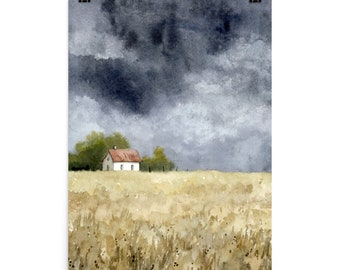The painting depicts a melancholic, wide-open landscape dominated by a dark, gloomy sky, suggesting an impending storm. The sky, filled with ominous gray and near-black clouds, forms the dramatic focal point of this portrait-mode watercolor painting. Below this turbulent sky lies a barren field of golden and beige grass that stretches out to a tiny countryside house in the distance. This minimalistic house, rendered with cream-colored walls and a brownish-red roof, features two side windows, a door, and a chimney. Sparse, basic fencing surrounds the house, adding to the scene's sense of isolation. Flanking the house are a few green trees, their simplicity mirroring the overall emptiness and surrealistic aura of the setting.